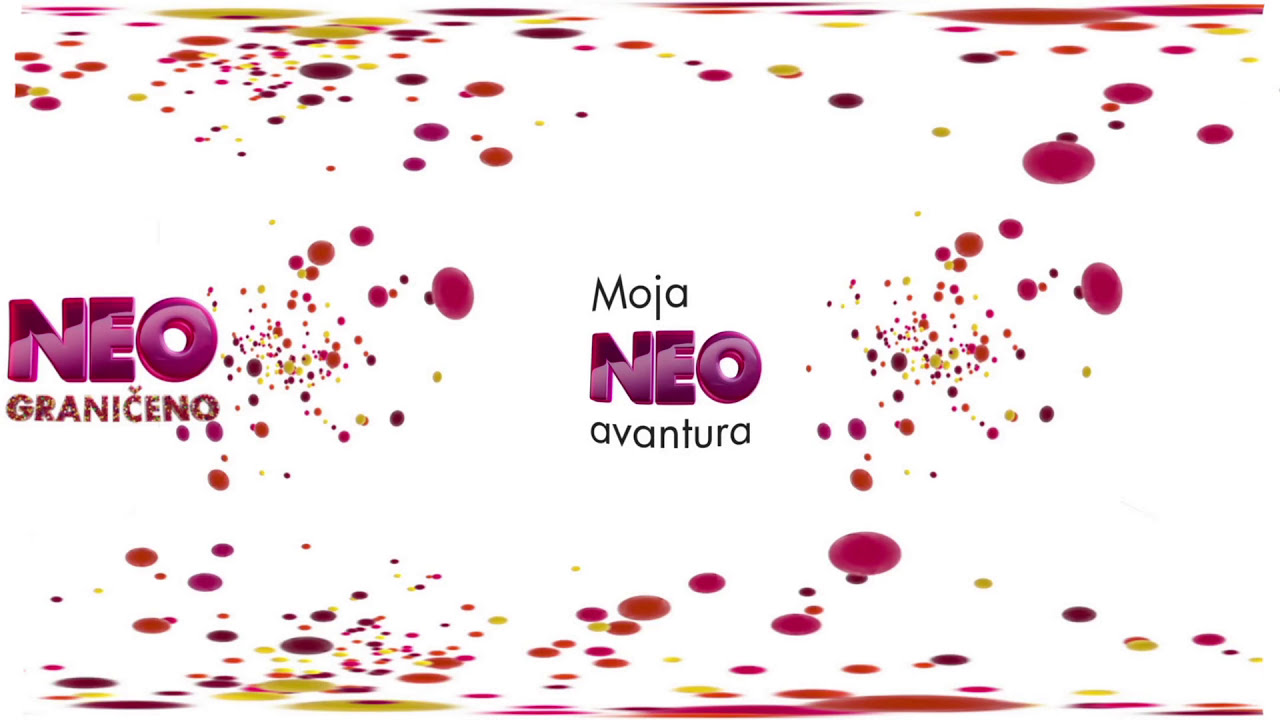The image features a predominantly white background interspersed with clusters of circles and splotches of various sizes and colors, including pink, maroon, yellow, and orange. At the top of the image, there are numerous colored circles, and these same types of circles appear throughout the image, forming distinct patches on the left and right-hand sides, as well as a band of circles across the bottom, mirroring the top. The text is prominently featured, with the phrase "NEO-GRANICENO" in pink and purple lettering on the left-hand side. In the middle, "MOJA" is written in black, followed by "NEO" in bold purple bubble letters beneath it. Below these, in black lettering, is the word "AVANTURA". The overall composition is a scattering of colorful dots against a stark white background, focusing on the colorful circles and central text elements.